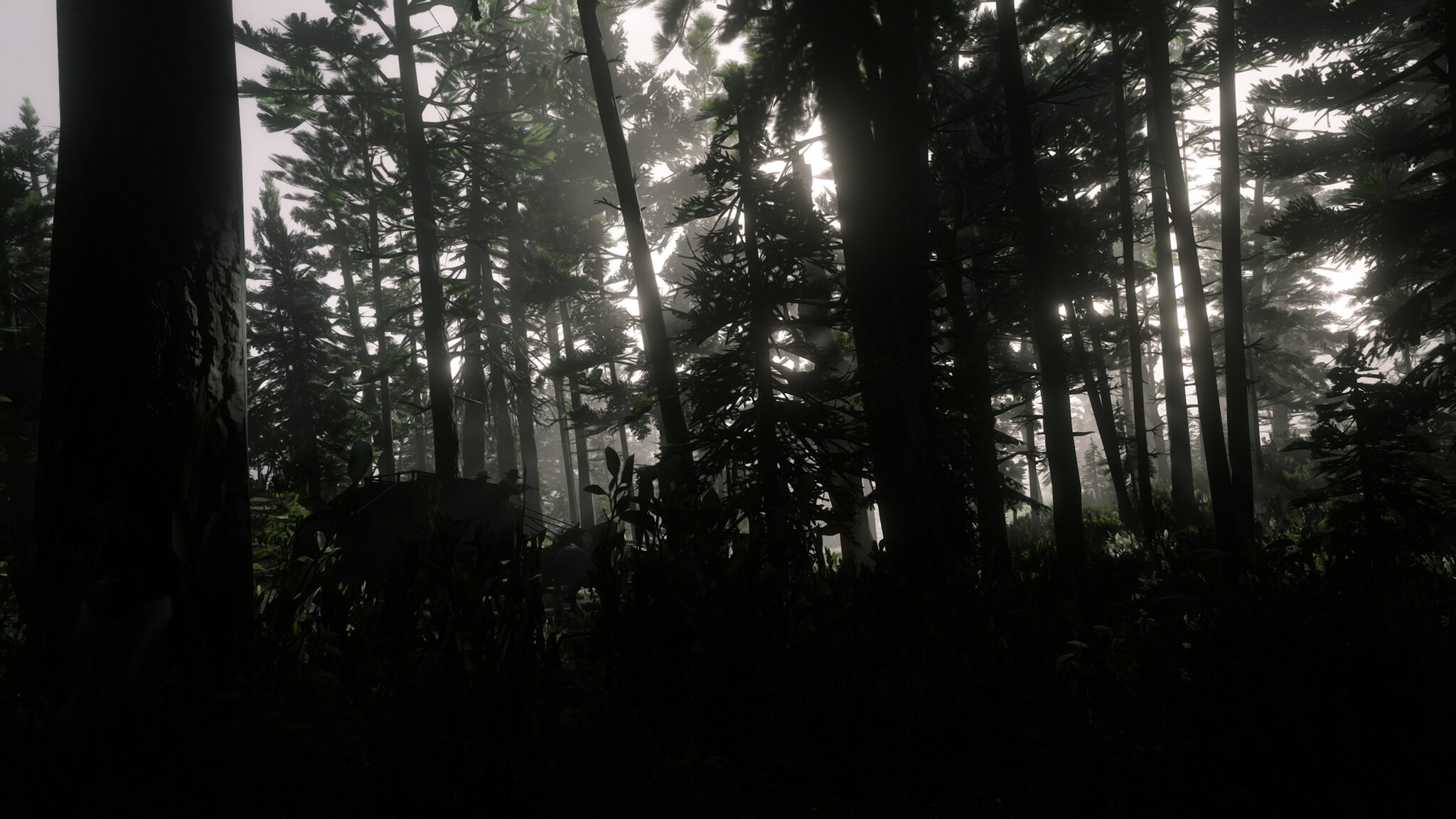In this photograph, we are presented with a dusky view of an enigmatic woodland. The scene is veiled in darkness, casting an almost eerie atmosphere. The bottom third of the photo is engulfed in blackness, obscuring any details that might lie beneath. Dominating the left side of the image is a very thick tree trunk, its surface appearing as dark as the night, ascending straight upwards and blending into the shadowy background.

The rest of the frame is filled with an array of slender tree trunks, rising vertically with no branches or foliage to break their stark outlines. Among these, a denser, darker trunk commands the center, its presence prominent and mysterious. Interspersed within the scene, a few fir trees can be vaguely discerned, their silhouettes adding to the forest’s dense texture.

In the upper right corner, the photograph hints at a broader environment with the partial appearance of fir tree branches extending from the right edge. The canopy above is sparse, allowing fragments of a gray sky to peek through the gaps between the trees. This diffused light illuminates the right side of the woodland slightly more than the left, adding a subtle gradient to the otherwise somber scene.